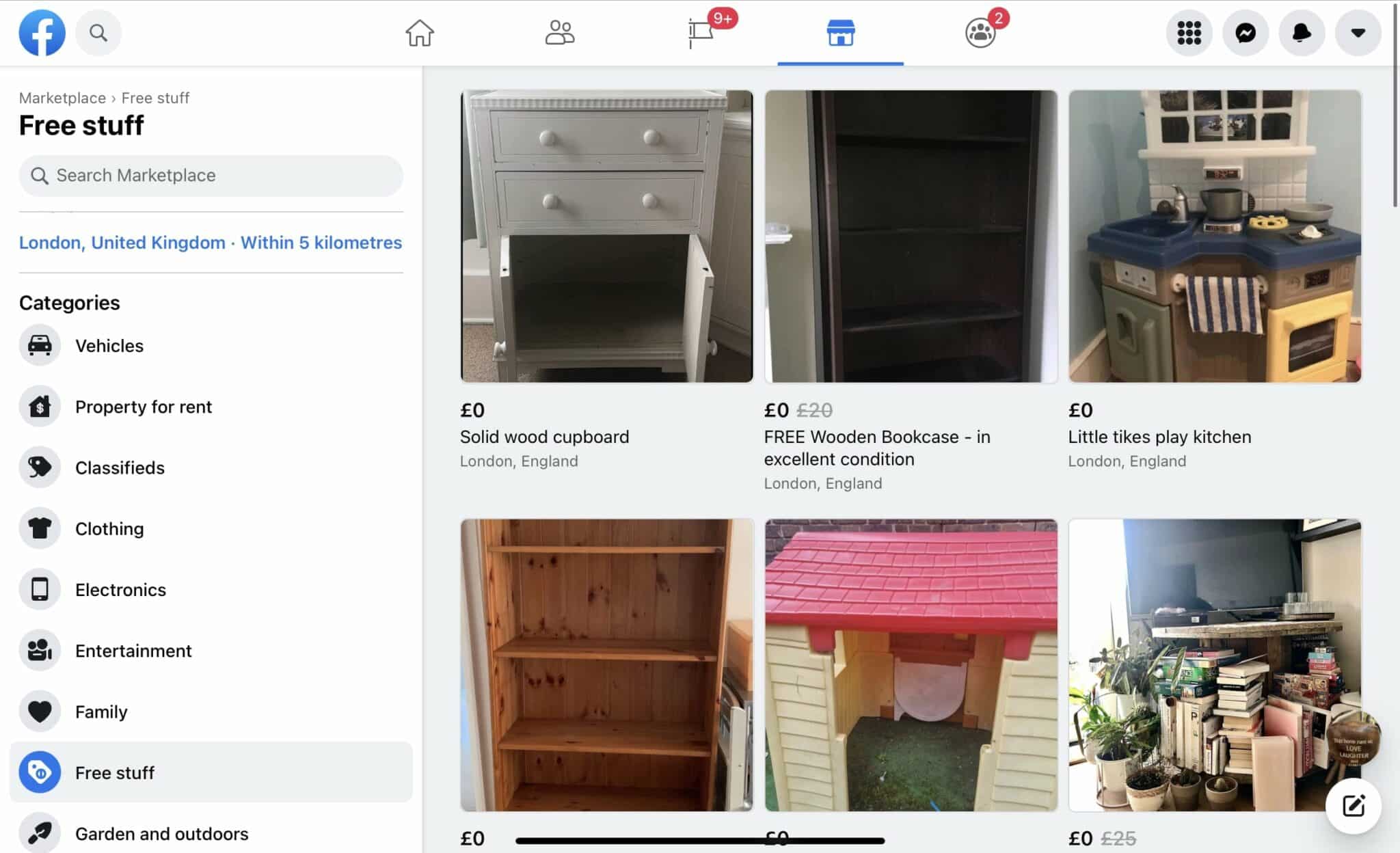This image is a detailed screenshot of a computer screen displaying the Facebook Marketplace interface. The recognizable blue circle with a white "F" logo is positioned in the top left corner of the screen. Directly below it is a row with various clickable icons: a home symbol, people symbol, notification symbol showing nine notifications, and a highlighted Marketplace symbol. The fourth icon, representing groups, indicates two notifications.

On the right side of the screen, there are additional functional elements such as a search button and other navigation options. The main section of the screen shows Facebook Marketplace with a prominent left-hand column highlighting "Marketplace Free Stuff" in bold text. Below it is a search bar, and a location detail indicated by a hyperlink stating "London, United Kingdom within 5 kilometers," which can be adjusted. Further down are categorized links including "Vehicles," "Property for Rent," "Classifieds," "Clothing," "Electronics," "Entertainment," "Family," "Free Stuff," and "Garden & Outdoors."

The right side of the screen displays thumbnail images of various items available in the "Free Stuff" category on Facebook Marketplace. The top left image depicts a small nightstand. The center image shows a bookcase, while the top right image displays a Little Tikes play kitchen. The bottom left image features another bookshelf. The bottom center image appears to be a children's plastic playhouse. The bottom right image shows a table cluttered with books and plants, making it unclear what is specifically being offered for free.